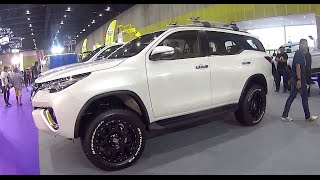This image, taken in a low-resolution, blurry, landscape orientation, depicts a white SUV, likely a CRV, prominently displayed at a car show. The photo is small, making intricate details difficult to discern, but the SUV, set at a diagonal angle from left to right, features four doors, black tires, and a gray roof rack suitable for luggage or bicycles. Its modern, pointy headlights add to the vehicle's sleek appearance. Indistinguishable branding is noted due to the car's positioning. The setting is a large indoor space, with gray walls, a dark black ceiling, light gray floors, and three rows of lit lights canopying the venue. People wander around, inspecting various exhibits, with more individuals clustered on the image's right side and behind the SUV, suggesting the lively atmosphere of a convention or car show. The image is bordered by thin black lines at the top and bottom, framing the scene.